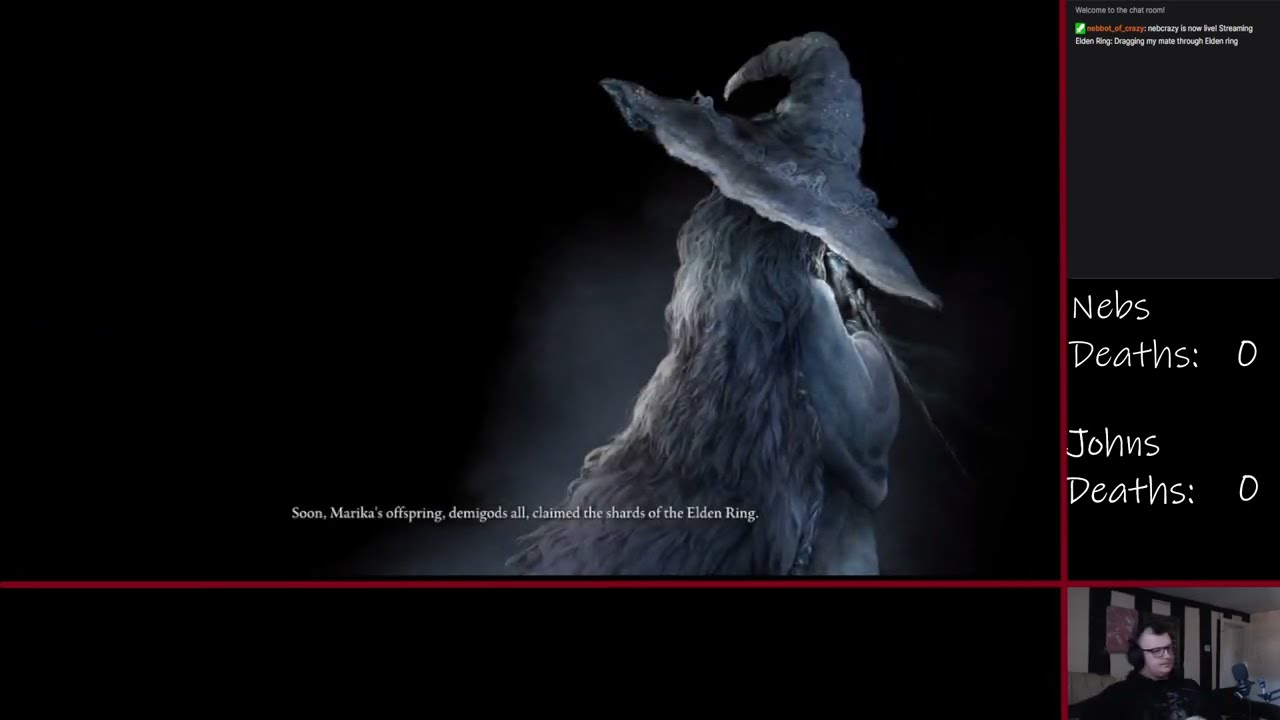The image appears to be a screen capture from a live stream of the video game "Elden Ring." Dominating the central portion of the frame is a hand-drawn style depiction of a faceless witch. She stands with her back to the viewer, sporting long, flowing bluish-gray hair and a large witch's hat, similarly colored in shades of gray. She also appears to be wielding a wand in the center-right of the image. The background is an ominous black, with wisps of smoke or mist that silhouette the witch.

At the bottom-center of this central image, white text reads, "Soon Marika's offspring demigods all claim the shards of the Elden Ring," providing context from the game. On the right side of the frame, there is a live-stream chat, though the messages are unreadable. Just below the chat, white text on a black background tracks the streamers' progress, displaying "Neb's Deaths: 0" and "John's Deaths: 0."

In the bottom-right corner, a picture-in-picture shows the streamer, a white man wearing glasses and large headphones. He appears to be in his room, sitting in front of a wall marked by vertical black and white stripes.